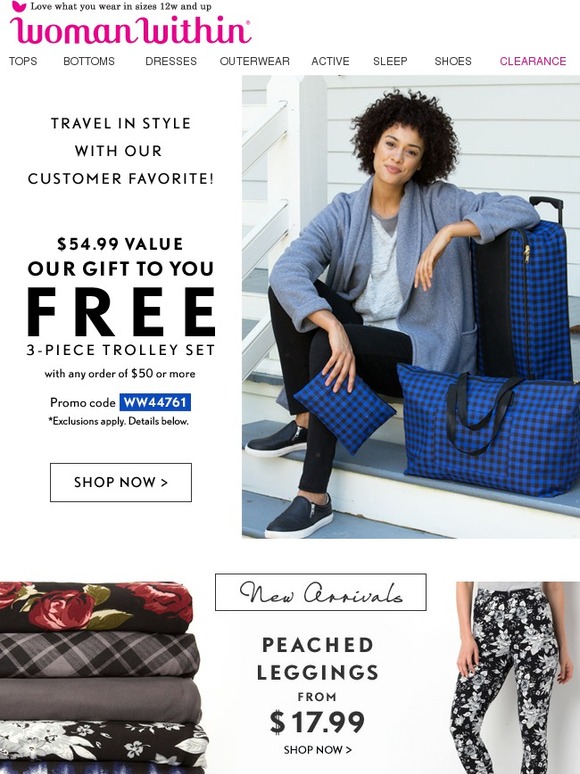This image depicts a promotional webpage for the brand "Woman Within." At the top of the page, the brand name is displayed in purple along with their slogan, "Love What You Wear," which caters to sizes 12W and up. The navigation bar features various categories including Tops, Bottoms, Dresses, Outerwear, Active, Sleep, Shoes, and Clearance.

The advertisement highlights a special offer, inviting customers to "Travel in Style with Our Customer Favorite $54.99 Value.” Shoppers are gifted a free three-piece trolley set with any purchase of $50 or more, using the promo code WWW44761. Notable small print mentions that exclusions apply and details can be found below. A "Shop Now" button is prominently displayed for easy access.

To the side, there is an image of a woman seated on steps, showcasing the advertised luggage set. She carries a duffel bag, a purse, and a wheeled suitcase adorned with dark blue squares. Her attire includes a gray jacket and black pants, emphasizing a chic yet comfortable travel outfit.